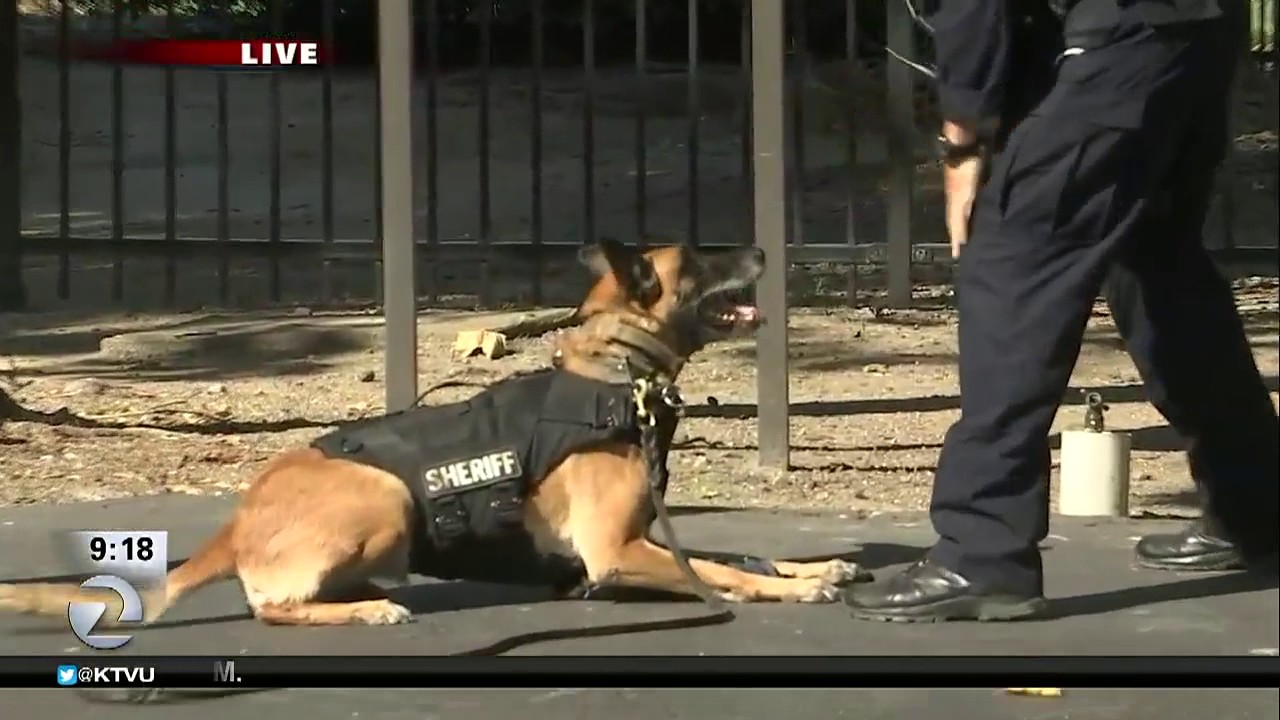The image shows a live broadcast screenshot from the KTVU news channel at 9:18 PM featuring a scene with a sheriff's office. In the upper-left corner, there's a red bar with white text indicating "live." The lower-left corner displays "9:18," "Channel 2," and the Twitter handle "@KTVU." Central to the image is a German Shepherd police dog, identifiable by its light tan coat with dark black markings on its ears, face, and mouth, which is open with its pink tongue hanging out. The dog is sitting down and is equipped with a black vest that has a white tag reading 'sheriff' on the side, and a black leash clipped to its harness, laying on the ground. To the right, we see the legs of a police officer in a dark navy blue or black uniform and black boots. The officer appears to be involved in training the dog.